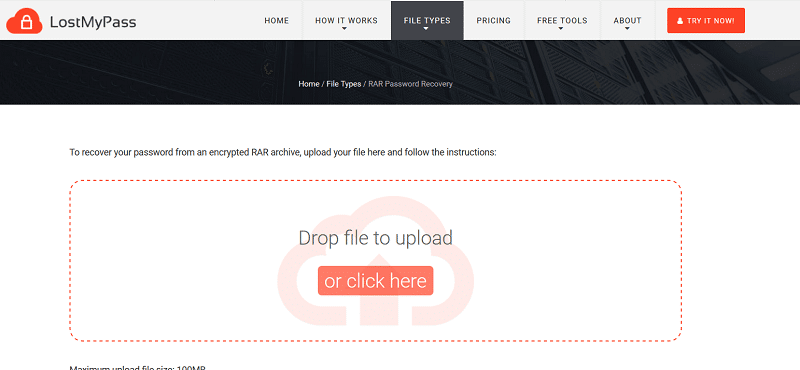The top section of the web page prominently features the name "Lost My Pass" positioned on the top left. Adjacent to the name is an orange cloud icon with a white lock symbol inside. The navigation bar at the top includes the tabs: Home, How It Works, File Types, Pricing, Free Tool, and About. The currently selected tab, "File Types," is highlighted with a black background and white text, unlike the grey background and black text of the other tabs. An orange "Try It Now" button is located at the top right.

Below the navigation bar, breadcrumb text reads "Home > File Types > RA Password Recovered," set against a black background featuring an image of buildings, with the text in white. Further down, the background shifts to white with black text instructing users to recover their password from an encrypted RA archive by uploading their file. The instructions are accompanied by a dotted orange outline box in the center of the page, which prompts users to "drag file to drop here." An alternative orange button labeled "or click here" is placed within the dotted box. A red cloud watermark is subtly displayed in the background. At the bottom left corner, text indicates a maximum upload file size of 100 megabytes.